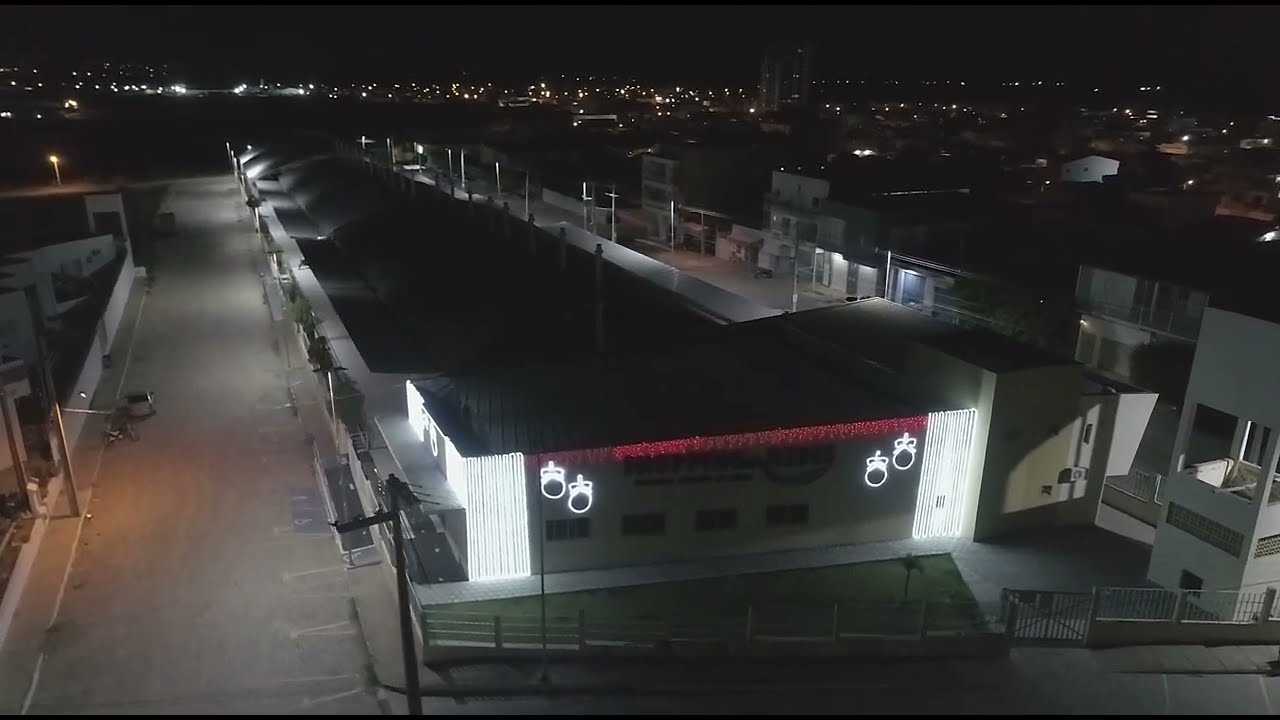This nighttime photograph captures a long, flat-roofed building, possibly a warehouse or dock, illuminated by bright white lights that line the entire structure. The roof is adorned with a string of red lights, giving it a festive appearance. In the foreground, you can see what appear to be ring-like images or possibly decorations, with two on either side of the building's corners. The scene is further defined by a well-lit sidewalk running alongside the building and multiple streetlights that illuminate the area. Beyond this structure, more buildings can be seen on the right, contributing to what seems to be a small-town industrial or business district. In the distance, the landscape is dotted with city lights, indicating a suburban area devoid of large skyscrapers but filled with smaller, flat-roofed buildings. The overall ambience suggests a quiet, industrial part of town, with roads encircling the illuminated structure.